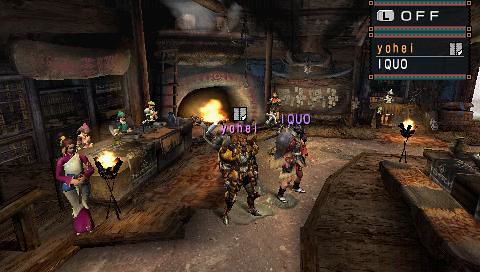This screenshot appears to be from a multiplayer video game. The scene is set in a dimly lit, rustic tavern with heavy use of brown earth tones contributing to a notably Nordic aesthetic. Overhead, unique usernames rather than traditional character names can be seen, suggesting the multiplayer nature of the game. 

In the foreground, there are two characters, likely orcs or barbarians, clad in rugged-looking armor. Due to the small size of the characters in the image, finer details are difficult to discern. 

Off to the side, three men are seated at a wooden table, engaged in a likely conversation or activity. Beside them stands a woman who appears to be some kind of server or tavern worker. Her attire, while not authentic, displays clear East Asian influences, hinting at a blend of cultural elements within the game's design.